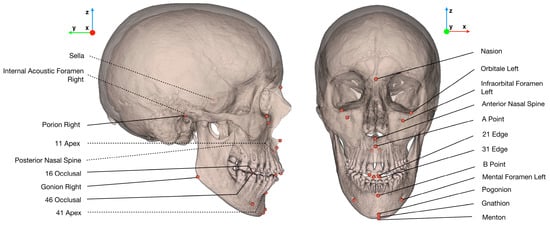This detailed anatomical illustration features two human skulls, presented in a style reminiscent of a textbook or postcard. The left skull is depicted in profile, with its front facing to the right. Key anatomical landmarks such as the top part of the skull, nasal cavity, teeth, and jaw are clearly visible. Surrounding this skull, various lines radiate to the left, each terminating with a label identifying specific skull components.

In contrast, the right skull is shown from a frontal perspective, allowing a clear view of the eye sockets, nasal cavity, and jaw with teeth. Similar to the left skull, this one also has lines extending from various red dots on its surface to the right, each line pointing to a descriptive label.

Both skulls are rendered in a pale white-gray color, with intricate details preserved to make them appear anatomically accurate. Additional features include a small graph in the upper left-hand corner, demonstrating axes marked X, Y, and Z, with horizontal green and vertical blue lines converging at a red dot.

Overall, this illustrative image serves as an educational diagram, precisely labeling various parts of the human skull with informative annotations, designed to aid in learning and understanding skull anatomy.